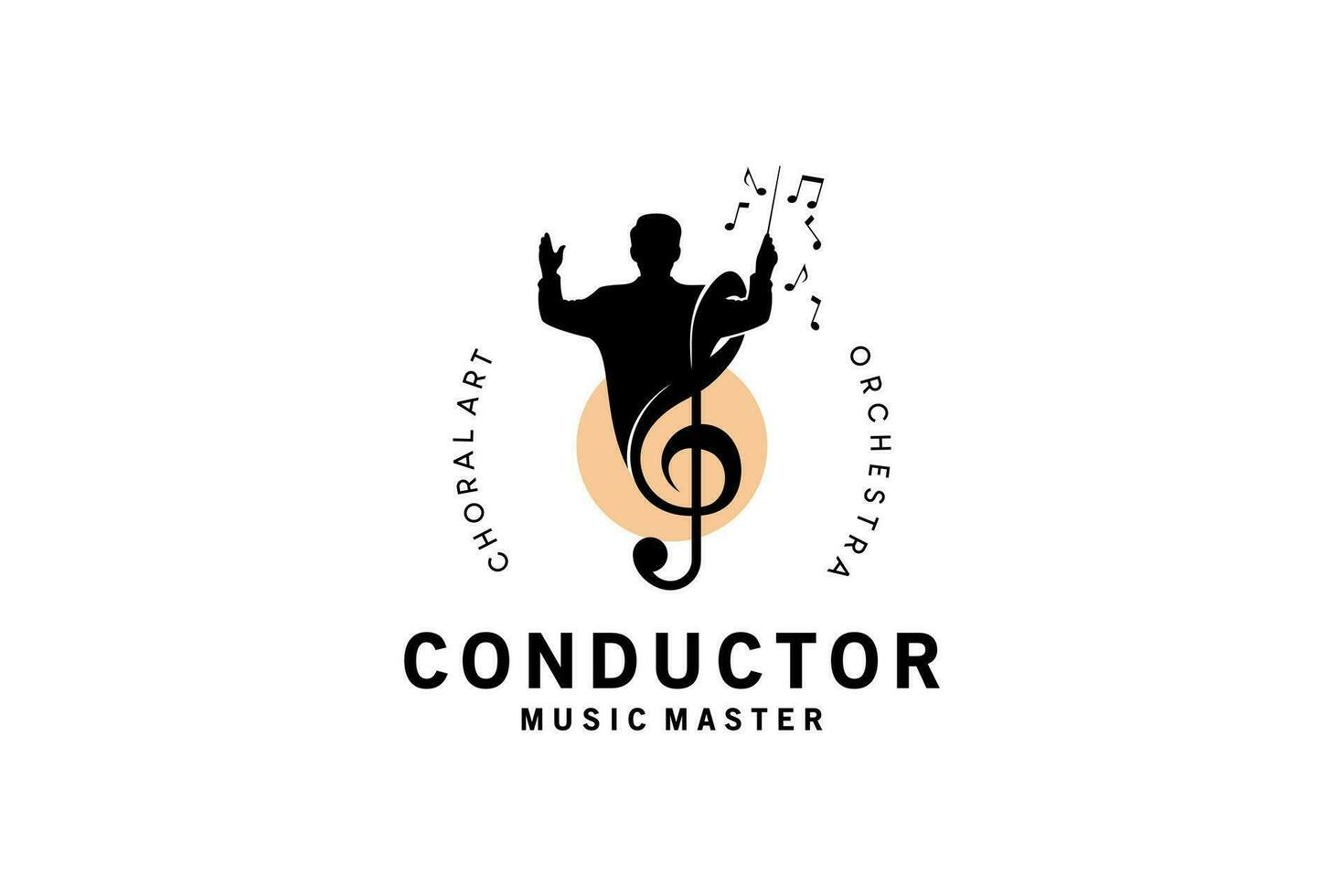This image serves as a detailed logo for a Choral Art program, potentially indicative of a school or art initiative. Set against a white background, the periphery of the logo features black text, forming a circular frame. On the left side, it reads "Choral Art," and on the right side, it says "Orchestra." Below these words, prominently centered in larger, capitalized black text, is the word "CONDUCTOR," with "Music Master" in a smaller font immediately beneath it.

Dominating the center of this circular logo is a silhouette of a conductor, rendered entirely in black. This figure stands in front of a smaller, light orange or tan circle, from which he emerges. The conductor is positioned from the back, with both arms elevated, and holds a baton in his right hand. Musical notes are depicted floating around the tip of the baton, emphasizing his dynamic movement. Additionally, a large musical note, resembling a treble clef, wraps around the conductor's right arm and extends down his back, adding an artistic flourish. His chest area forms into a V shape, mirroring the shape of the treble clef, thereby integrating musical elements seamlessly into the figure's design.